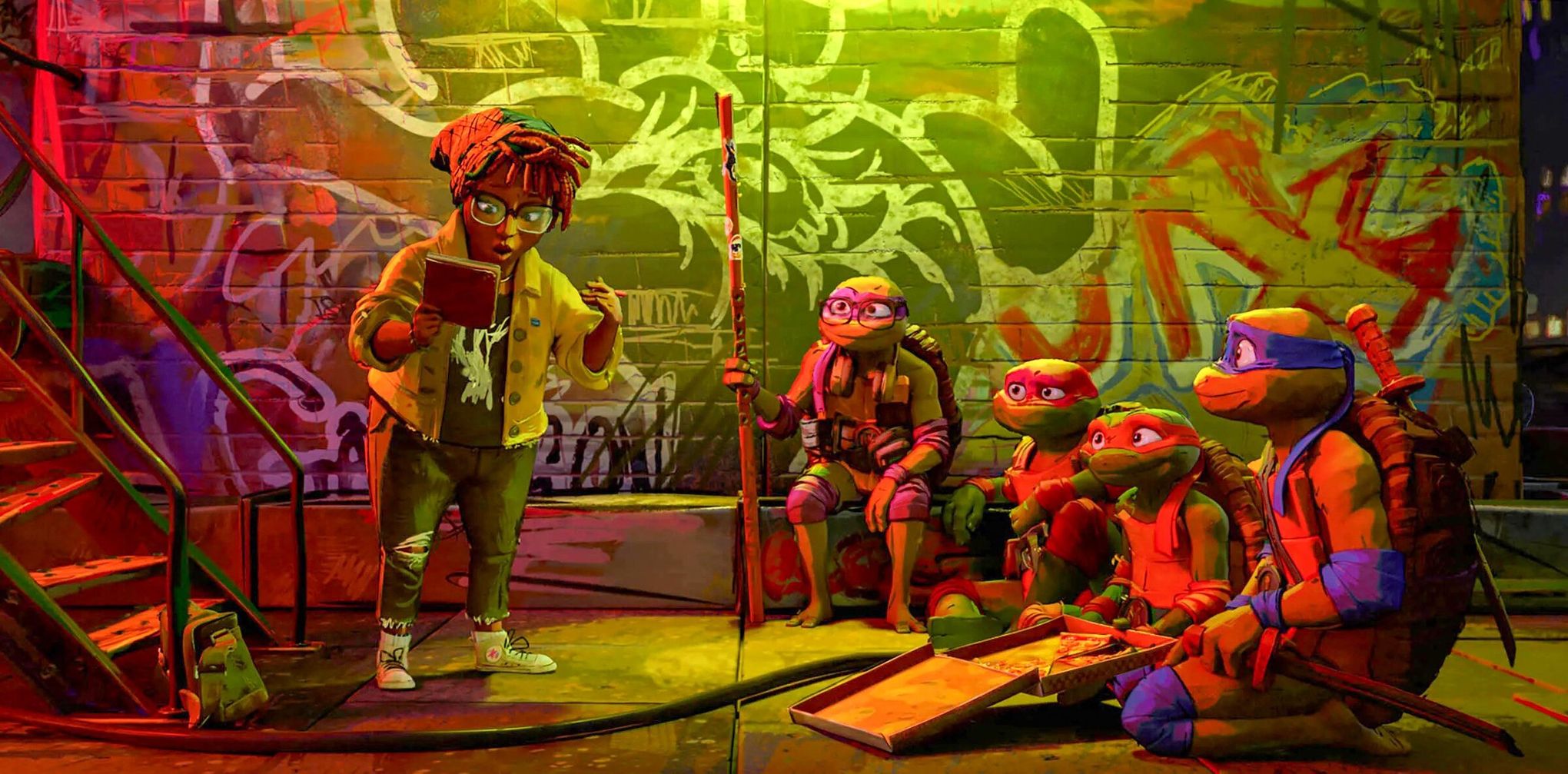This highly detailed animation-style image features the Teenage Mutant Ninja Turtles in their latest iteration, positioned against a vivid backdrop of graffiti-covered walls. The graffiti is an explosion of colors, characterized by a blend of bright pink and white on the left, a striking green center with white lines, and unreadable yellow letters outlined in red on the right. The scene is set outdoors, illuminated with intense green lighting while a rust hue subtly tinges the left side and the turtles themselves.

The Teenage Mutant Ninja Turtles, dressed in their iconic colored bandanas—purple, blue, red, and orange—are seated in a row on the floor, attentively looking at a woman standing before them. This woman, identified as April O'Neil, is depicted with short hair secured by a handkerchief, and she wears a long-sleeve yellow jacket paired with green pants and a green shirt. She is engrossed in reading from a book or pamphlet. Additional details include her glasses, ripped-knee jeans, sneakers, and a backpack placed on the stairwell next to her. 

In front of the turtles, identifiable by their character designs from the most recent Teenage Mutant Ninja Turtles movie, there's a nearly-finished pizza box with only a slice or two left. The vibrant and dynamic atmosphere reflects the modernity and energy of the latest film, presumably associated with actor Seth Rogen's involvement in the project released last year.